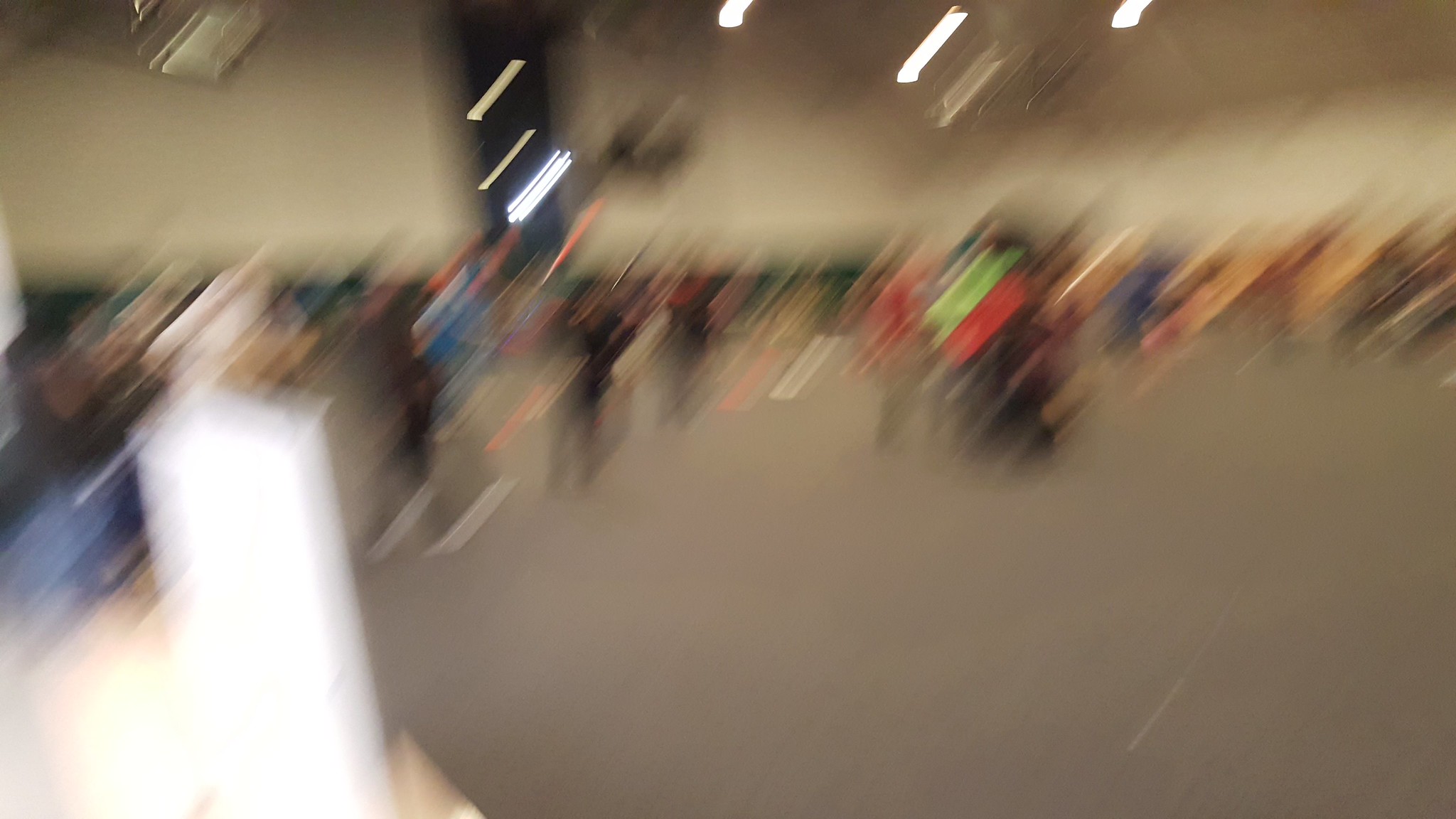This color photograph features a decidedly blurry, out-of-focus scene that appears to be intentionally crafted for special effects. Dominating the bottom half of the image is what seems to be a slate gray floor surface with some gradation and undertones of medium to light brown. In the lower left corner, a white, oblong, and vertical object can be vaguely discerned, though it remains indistinct due to the pervasive blurriness. The middle portion of the photograph, spanning from side to side, suggests a large crowd of people, indicated by a myriad of colorful clothing. Despite the lack of sharp detail, the colors stand out, including shades of turquoise blue, red, and various grays, both light and dark.